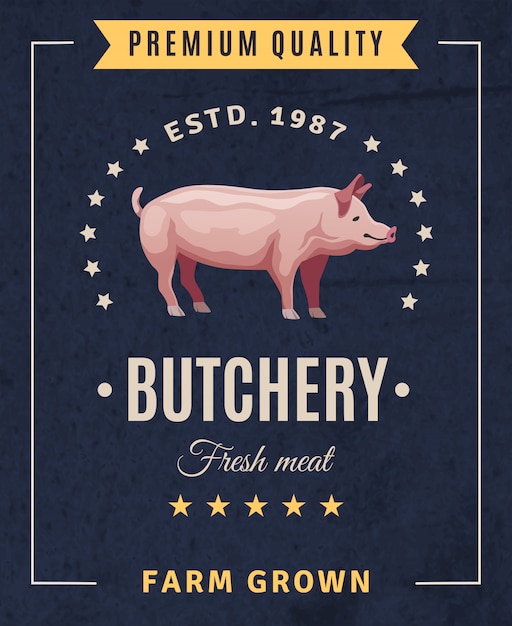This image features a graphic advertisement with a predominantly navy blue background and a white border. At the very top, a golden-yellow ribbon with navy blue, all-uppercase text states "PREMIUM QUALITY." Directly beneath it, in uppercase letters, the ad reads "ESTD 1987" accompanied by stars on the left and right. Central to the design is a graphic of a pig with pink ears, nose, and tail, facing right and appearing as if it might be smiling. Below the pig, in large white uppercase letters, is the word "BUTCHERY," followed by the phrase "FRESH MEAT" in cursive script. Further down, there are five gold stars, culminating at the bottom with the text "FARM GROWN" in large gold letters. The combination of these elements suggests an advertisement for a butcher shop emphasizing premium quality, fresh meat, and farm-grown products.